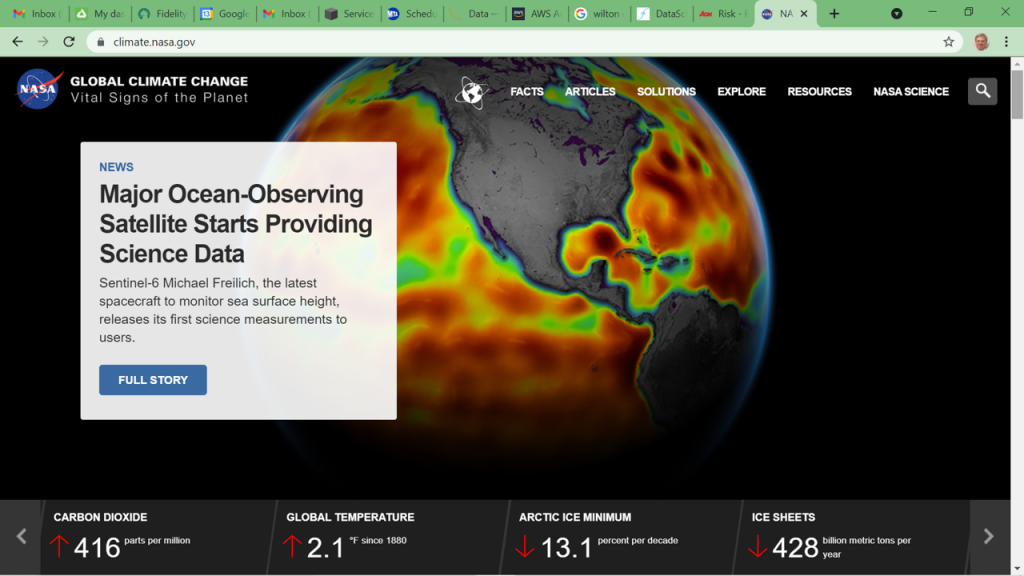A detailed screenshot of the NASA website focused on global climate change and the vital signs of the planet. The homepage prominently features a heat map of Earth, displaying color-coded temperature variations: red, yellow, and lime green areas indicating different temperature zones. The top-right corner showcases a bold navigation menu, with white, uppercase font reading: FACTS, ARTICLES, SOLUTIONS, EXPLORE, RESOURCES, and NASA SCIENCE. At the bottom of the screen, black metric bars present critical climate data, including carbon dioxide levels, global temperature, Arctic ice minimum, and ice sheets. On the left side, a white square highlights a news article titled "Major Ocean Observing Satellite Starts Providing Science Data," accompanied by a brief description and a clickable blue button for the full story. The browser reveals several open tabs, indicating multiple ongoing activities. The interface confirms usage of a Microsoft computer, discernible by the window management icons.